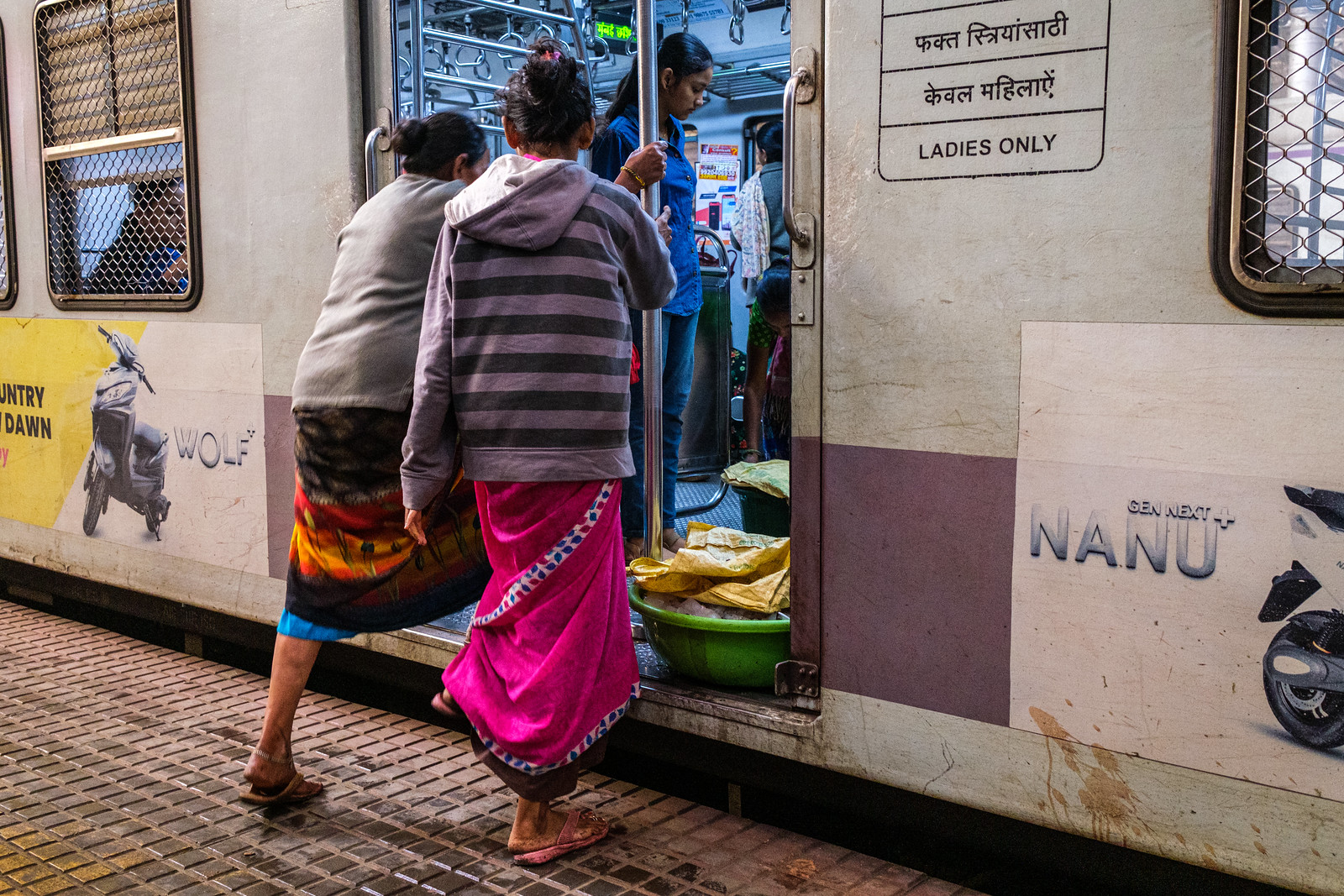In this image, two women are boarding a run-down bus, potentially in Mexico or Cuba. The bus is adorned with advertisements, including one that says "Wolf" and another that mentions "Not New." The bus features multiple windows and is surrounded by a fence-like structure. Inside, a person is seen holding a pole, reminiscent of subway railings. The women are dressed in colorful attire—one wearing a pink dress and flip-flops, and the other in a dress with shades of orange, red, and blue. The girl inside the bus is noted to be wearing a blue shirt. Additionally, a sign in Middle Eastern characters on the right side reads "Ladies Only," indicating a degree of segregation.